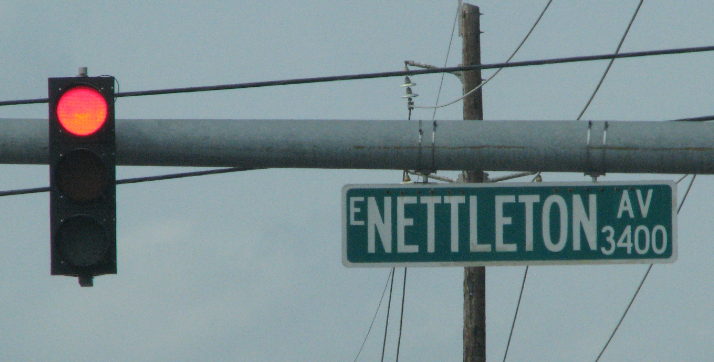A photograph taken on a gray, cloudy day captures a street scene featuring a metal pole and its attached fixtures. The pole, constructed from thick, grayish-silver metal, supports various elements. On the left side, a stoplight with a black metal frame displays a red light at the top, while the yellow and green lights remain unlit. Beneath the horizontal arm of the pole, a green street sign with white lettering reads "E. Nettleton Ave 3400." In the background, a network of black electrical wires crisscross both horizontally and perpendicularly across the image. Additionally, a plain brown telephone pole with metal attachments adds to the urban composition. The overall ambiance of the photograph is marked by the overcast sky and the intricate interplay of urban infrastructural elements.